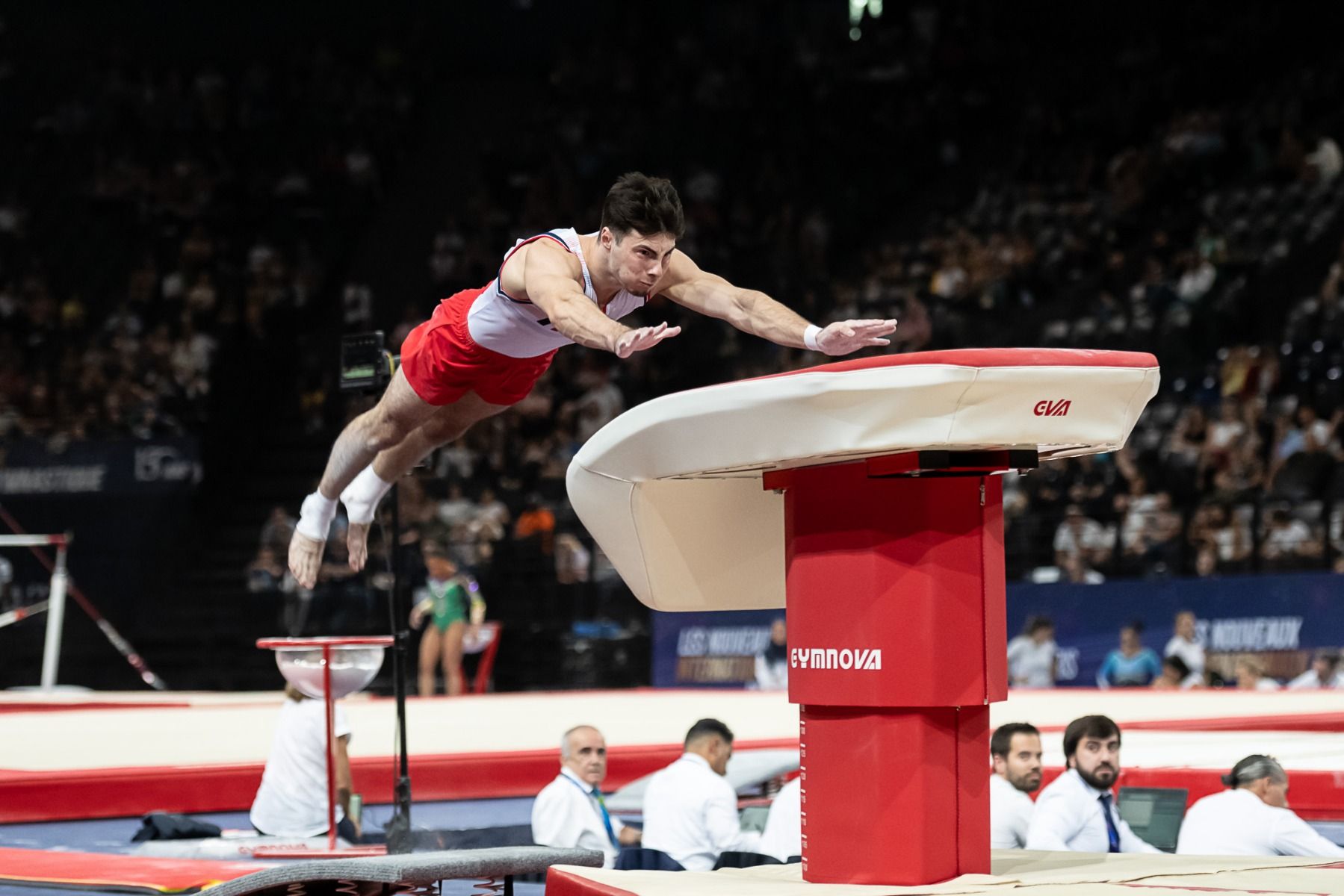At a bustling gymnastics sporting event, a male gymnast is captured midair, diving with outstretched arms onto a white apparatus with a red top and base, branded E-Y-M-N-O-V-A. He is Caucasian, of athletic build, with short dark hair, wearing a white tank top and red shorts, and has white tape around each ankle. Below him, several men in white shirts and ties, likely judges or officials, are gathered. The background features full bleachers with a blue barricade at the bottom, a crowd of spectators, and a faint netting, suggesting a large, possibly Olympic, arena setting. The scene is filled with an air of anticipation as the gymnast showcases his skill.